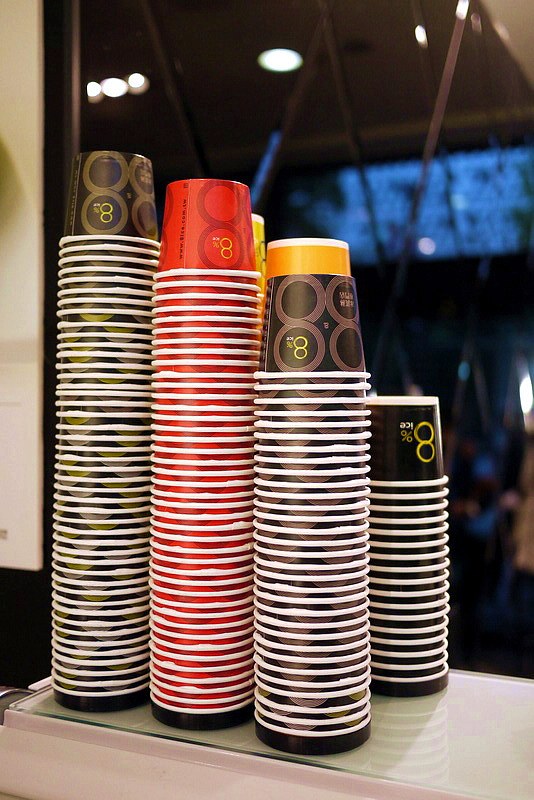In a brightly lit cafe, a variety of paper cups and bowls are meticulously stacked on a glass pane placed atop a white rectangular bar surface. Starting from the left, the first stack is the tallest, comprising slender bowls decorated with light brown circles and a gold number '8' within one circle. The second stack features similar bowls but in a striking red hue, adorned with dark red circles and a yellow letter 'B'. The third stack transitions to cups, which are gold at the bottom with a brown circular print around the top, each featuring an '8' in one of the circles. Behind these, slightly to the right, is a fourth stack of black bowls, prominently displaying a large number '8'. The background of the image hints at a typical cafe setting with overhead lighting and a visible menu board, adding context to the scene's coffee shop ambiance.